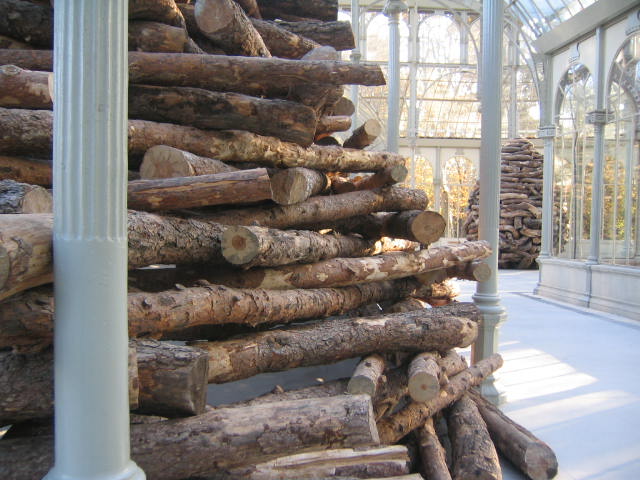The photograph captures the interior of a vast glass building, akin to a greenhouse, marked by extensive windows comprising its walls and ceiling. The architecture is supported by numerous gray or white pillars, which are narrow yet extend from floor to ceiling, suggesting they are structurally significant. The interior space is dominated by substantial piles of wood, prominently featured in both the foreground and background. These wood stacks are comprised of logs seemingly cut from small trees, each about 3 to 4 inches in diameter and ranging from 4 to 6 feet in length. The piles are meticulously arranged, some forming teepee-like structures that start broad at the base and taper to a peak, reaching an approximate height of 8 feet, towering over the space. The symmetry and repetition of the pillars and wood stacks create a harmonious yet industrial-like ambiance within this expansive glass enclosure. Through the glass walls, there is a subtle hint of the outside environment, offering a glimpse of trees beyond.